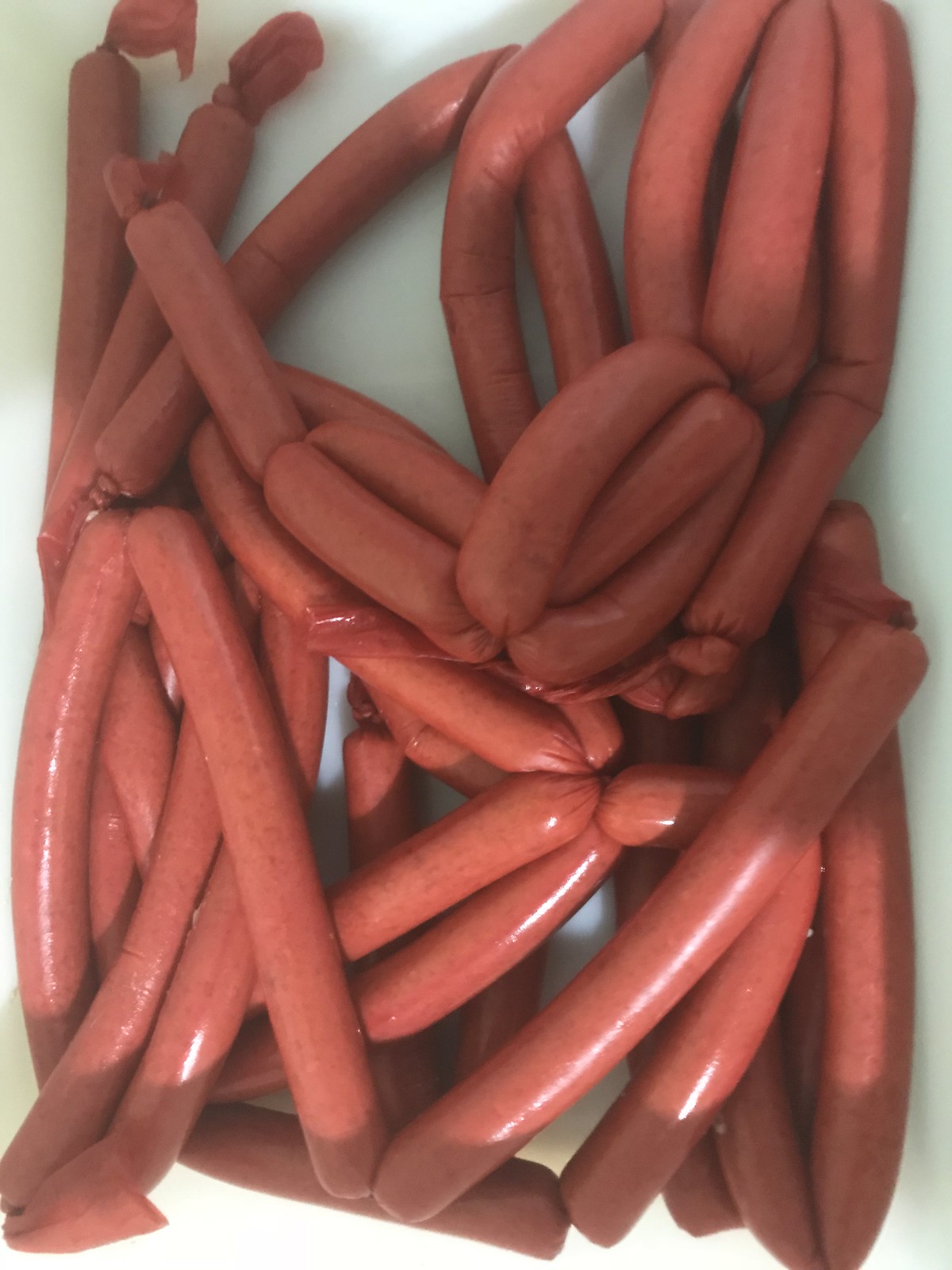This top-view photograph captures a chaotic pile of extra-long sausage links or hot dogs, all connected by their casings. The sausages, which are a typical reddish-brown color, are sprawled across a white background that appears slightly blue due to the shadows cast. Some sausages are doubled over, folded in half, and crossed over one another, while others are vertically placed at various angles. In the upper right-hand corner, a few sausages group together like a bunch of bananas. Towards the center, the sausages converge to form a knot-like structure, and at the bottom, two ends meet, resembling a V shape. These details collectively emphasize the messy, jumbled arrangement of linked sausages that cover the frame.